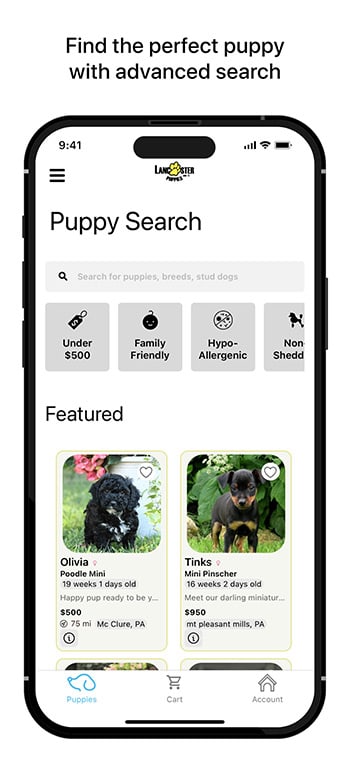The image features a graphic representation of a mobile phone screen showcasing an app for finding puppies. Above the mobile phone graphic, the title "Find the Perfect Puppy with Advanced Search" is displayed in bold black letters. 

The screen itself is detailed meticulously. In the upper left-hand corner of the phone screen, the time is shown as 9:41. On the upper right, standard indicators for battery, Wi-Fi, and cell signal strength are present. Centered at the top, a header reads "Lancaster Puppies" alongside a charming graphic of a yellow paw print.

Beneath this header, the phrase "Puppy Search" is prominently displayed in large letters. Below this, a search bar sits, ready for user input. Further down, the screen is divided into several light blue squares, each representing different search filters. From left to right, the filters are labeled: "Under $500," "Family Friendly," "Hypoallergenic," and a partially cut-off filter that appears to read "Non-Shedding."

Below these filters, a bold heading reads "Featured," introducing a section highlighting specific puppies. Two puppies are showcased with their respective details:

- On the left side, there is a small black puppy with the details: "Olivia, Poodle Mini, 19 weeks, 1 day old, $500, 75 miles away, McClure, PA."
- On the right, a brown and black puppy named Tinks is featured with the description: "Tinks, Miniature Pinscher, 16 weeks, 2 days old, $950, Mount Pleasant Mills, PA."

This detailed layout provides a user-friendly interface for finding and selecting puppies based on various preferences and characteristics.